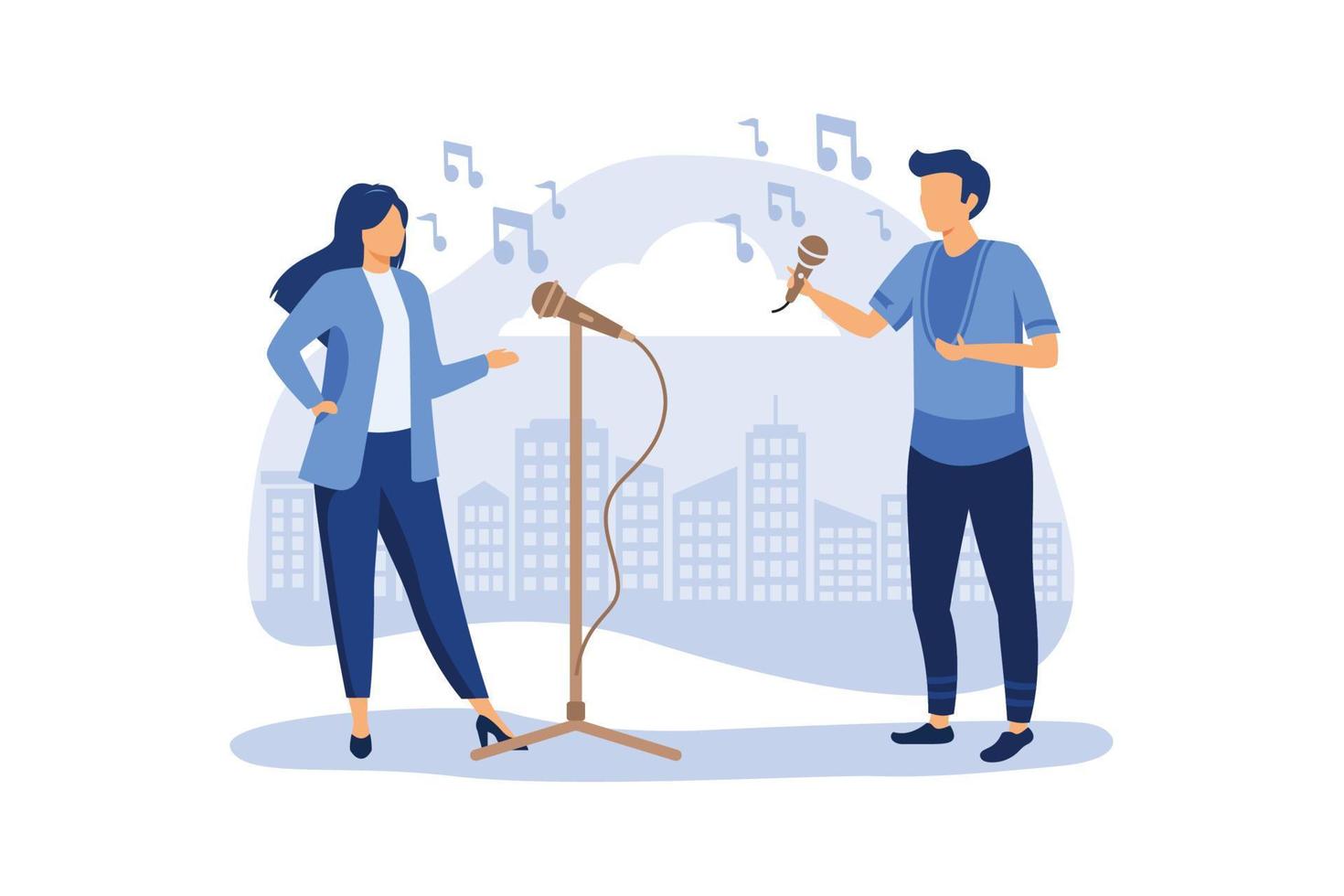The image is a clipart-style graphic featuring a man and a woman singing into microphones, both dressed in various shades of blue. Their faces are blank, lacking any defined features like eyes, nose, or mouth. The woman, positioned on the left, is wearing a blue jacket with a light blue top, darker blue pants, and blue high heels. She sings into a microphone mounted on a stand in front of her. The man, on the right, wears a blue patterned short-sleeve t-shirt, dark blue pants, and possibly very dark blue shoes. He holds a gold-colored microphone in his right hand, facing the woman. Both have dark blue hair, matching the predominantly blue theme of the image. They stand on a light blue surface, with a light blue-gray background that features a city skyline within a bubble. Scattered throughout the background are white clouds and floating blue music notes, enhancing the musical ambiance of the scene.